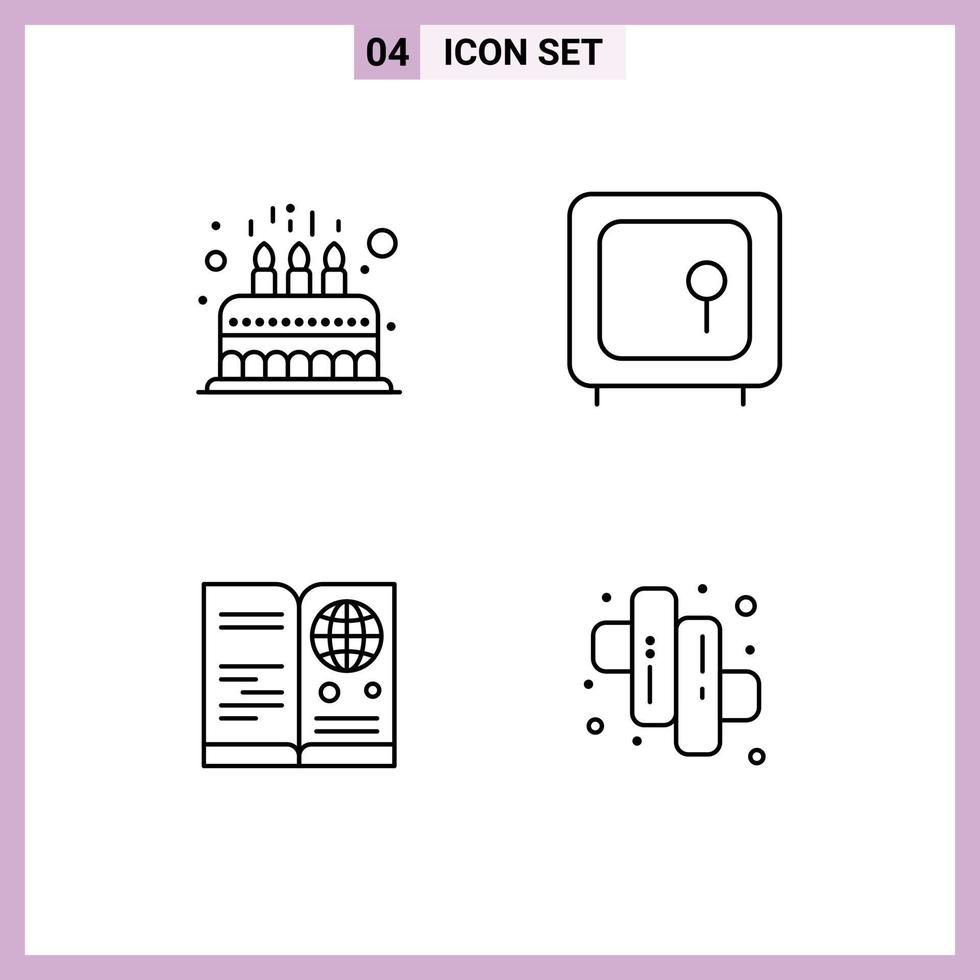The image is a black and white line drawing of an icon set, labeled "04 icon set" at the top in black text. The outline of the image is light purple, resembling lilac. The icons are arranged in a 2x2 grid, with two icons on the top row and two on the bottom row.

Starting from the top left, the first icon depicts a birthday cake with three candles. Lines above the candles suggest flames. To the right of the cake is an old-school TV set, characterized by a large screen in the center, a circular dial on the right side, and standing on two legs.

On the bottom left is an open book icon, featuring lines on both pages to represent text, and a picture of an orb, likely representing Earth, on the right page. The bottom-right icon consists of two vertical rectangles overlapping two horizontal rectangles, with various lines and dots, resembling a stacked geometric shape.

The overall aesthetic is minimalistic, consistent with typical iconography using black and white colors and clean, simple lines.